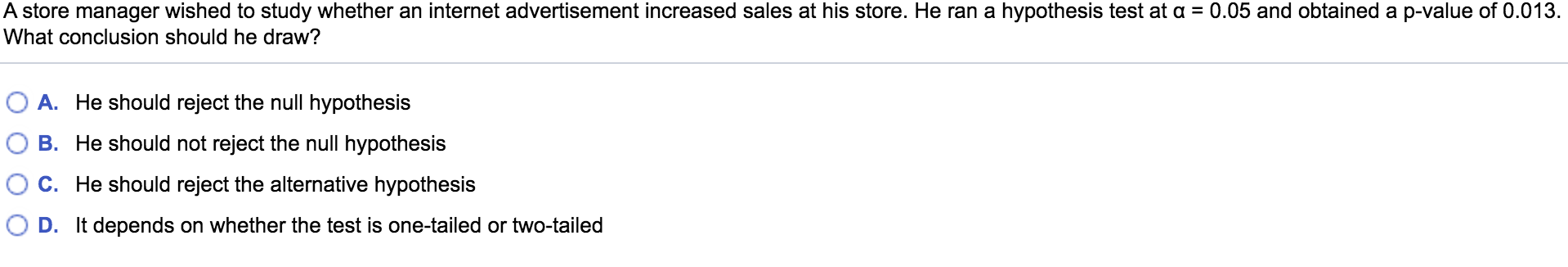A store manager seeks to determine if an internal internet advertisement has led to an increase in sales. He conducted a hypothesis test with a significance level of α = 0.05 and obtained a p-value of 0.013. Based on the results, what conclusion should he draw? Below the question, separated by a faint grey line, are multiple-choice answers listed vertically, each marked by an open circle and capital blue letters followed by periods:

A. He should reject the null hypothesis.
B. He should not reject the null hypothesis.
C. He should reject the alternative hypothesis.
D. It depends on whether the test is one-tailed or two-tailed.

There are no additional descriptions, links, or visuals accompanying this content.